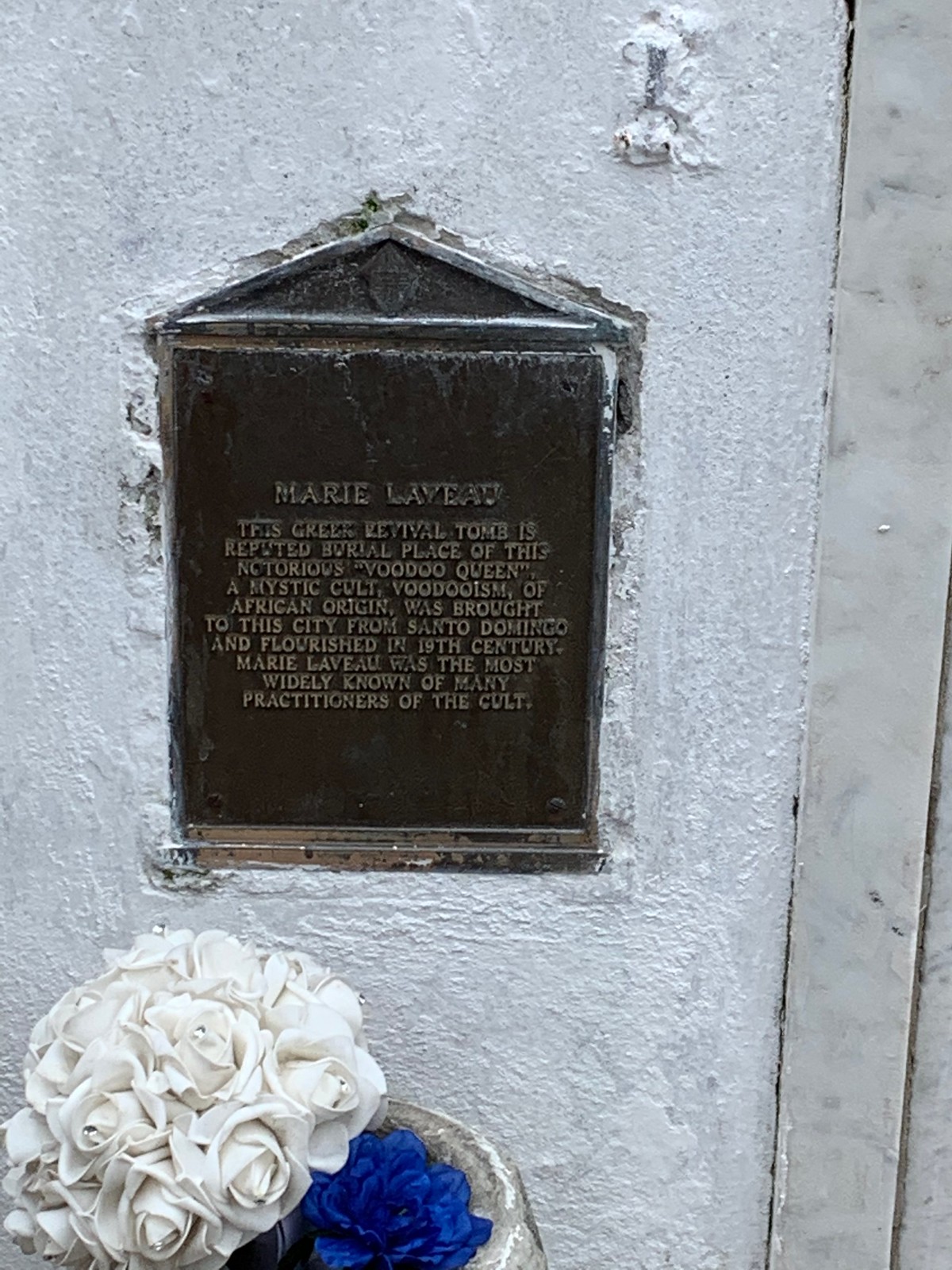The image is a bright, daytime, color photograph set against a historical white stucco wall, likely the exterior of a mausoleum. The central focus is a bronze, rectangular plaque with a triangular top, adorned with gold, slightly discolored, raised lettering. The plaque reads: "Marie Laveau. This Greek Revival tomb is the reputed burial place of the notorious Voodoo Queen. A mystic cult, Voodooism, of African origin, was brought to this city from Santo Domingo and flourished in the 19th century. Marie Laveau was the most widely known of the many practitioners of the cult." The plaque is positioned slightly to the left of center. At the bottom of the image, two clusters of blue and white roses are visible, adding a splash of color to the scene. This photo, characterized by representational realism, captures the essence of the historical and mystic aura surrounding Marie Laveau’s memorial.